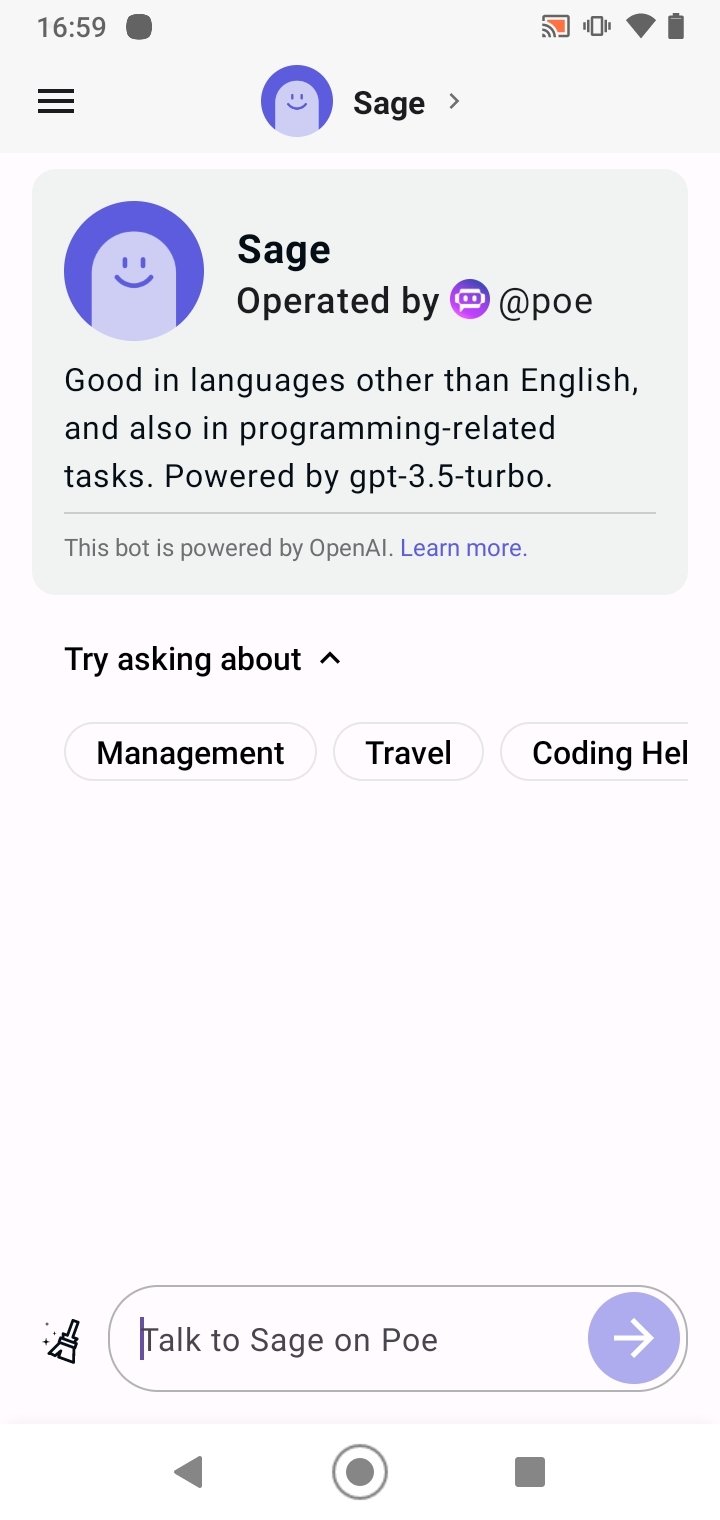The image displays the interface of an AI-powered chatbot called "Sage." The elements in the interface include the following:

- **Time Display:** Shows 16:59.
- **Status Icons:** Includes a vibrating phone icon, a Wi-Fi signal indicator, battery level, and three lines indicating options or settings.
- **Bot Identifier:** A blue circle accompanied by the name "Sage," suggesting the bot is operational.
- **Sage Details:** Sage is described as being proficient in languages other than English and capable of handling programming-related tasks.
- **Technical Specification:** The bot is powered by OpenAI's GPT-3.5 Turbo model.
- **Additional Information:** "Learn more" link hinting at further details about the bot's capabilities.
- **User Prompt Suggestions:** Suggests that users can ask about management, travel, and coding.
- **Interaction Instructions:** Includes a "Talk to Sage" prompt with an arrow pointing to the right, indicating further interaction options.
- **Navigation Elements:** A left arrow, a dot within a circle, and a gray square for additional settings or navigation.
- **Ad Confirmation:** A mention that it is an advertisement for an AI chatbot.

The overall image appears to be an advertisement promoting the Sage AI chatbot, highlighting its functionalities, technical specs, and user guidance for interactions.